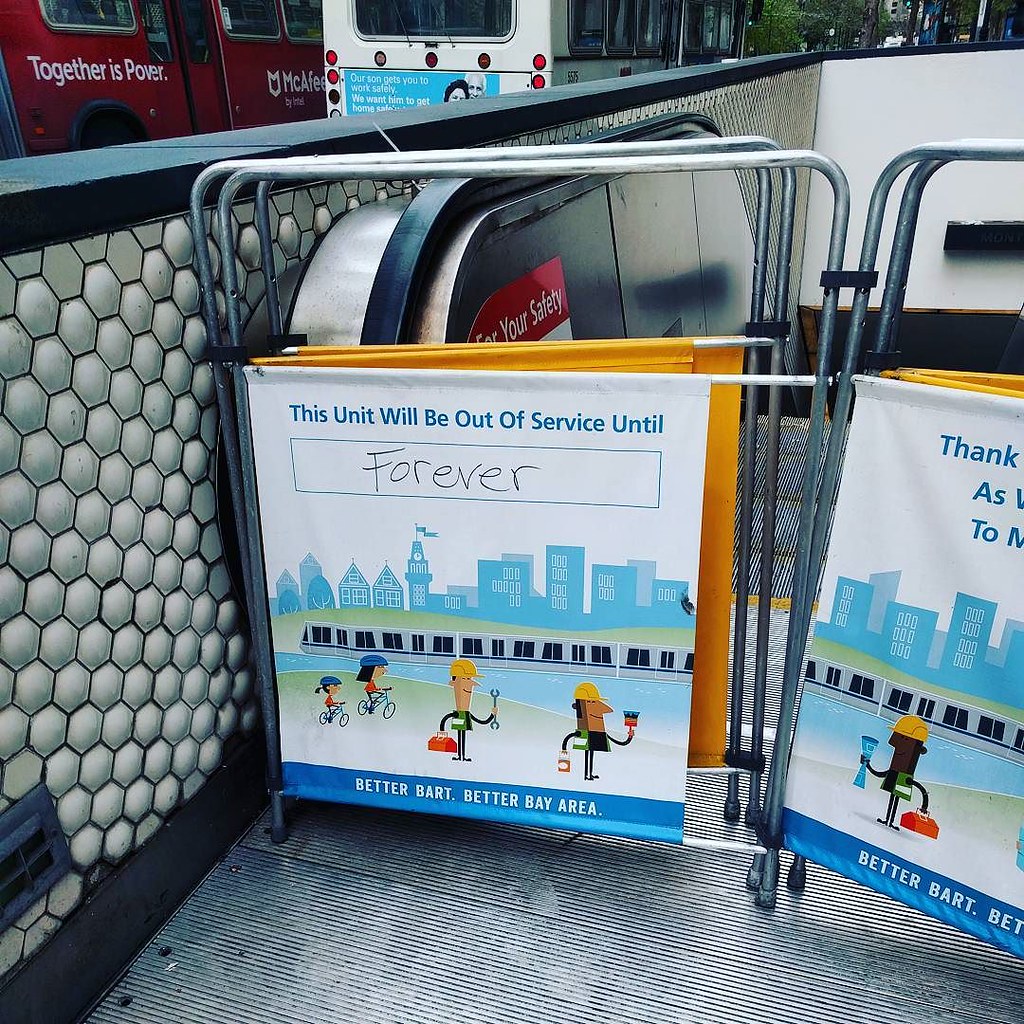The image depicts a bustling urban scene where a city appears within a larger cityscape. In the upper left corner, two buses are visible—one red and one white, each adorned with various advertisements. The central focus of the image is an out-of-service escalator, cordoned off by metal barriers featuring a prominently displayed sign. This sign announces in marker that "this unit will be out of service until forever" and bears the slogan "Better BART, Better Bay Area" at the bottom. The sign also includes a detailed illustration featuring a blue city skyline, a tram, water elements, and cartoon figures including cyclists and workers equipped with tools like a wrench and a paintbrush, one in a yellow hard hat. To the right of the image, portions of street signs, traffic lights, trees, and buildings are visible, enhancing the urban atmosphere.